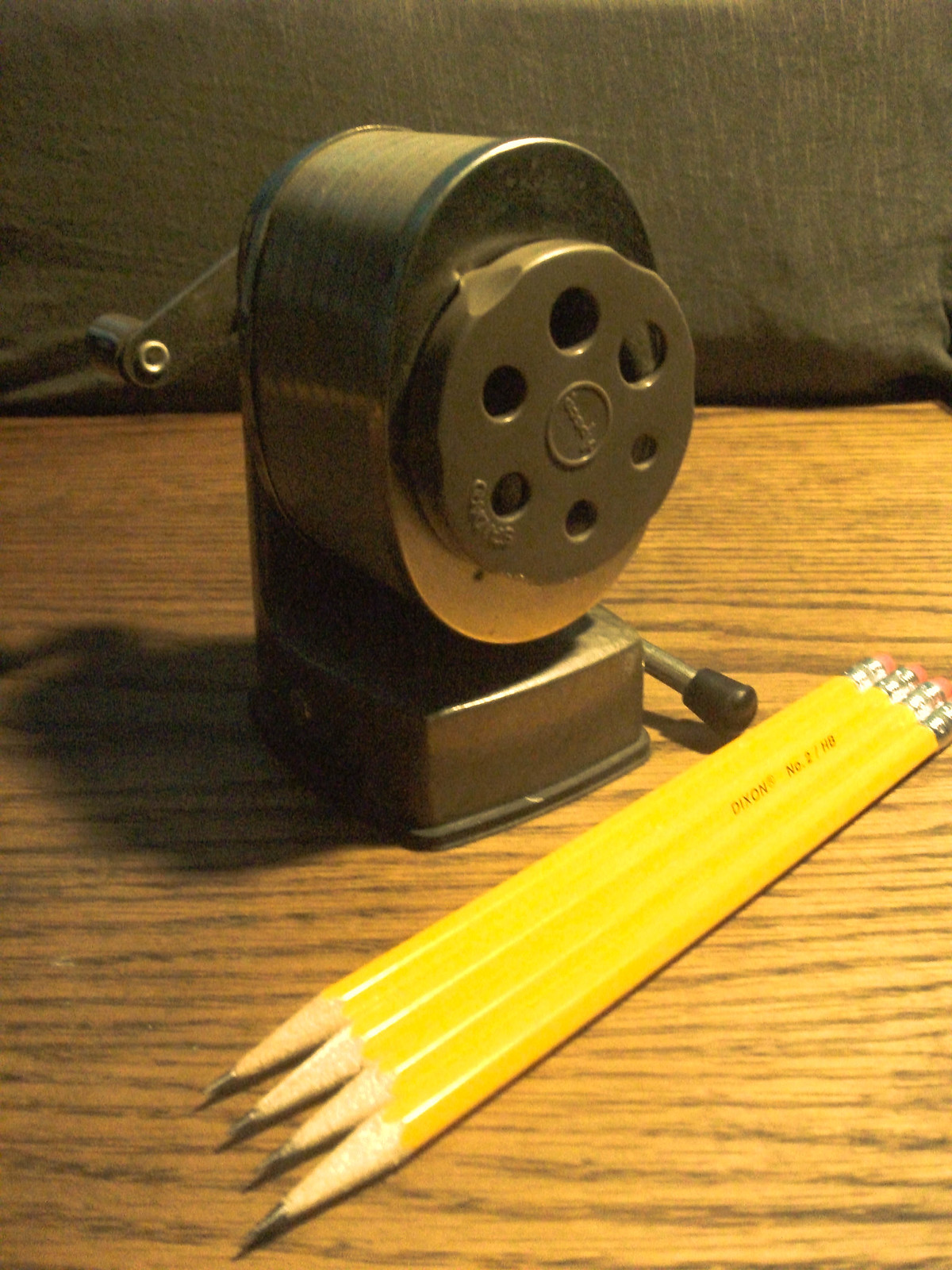In the center of this indoor color photograph is an old-time, metal pencil sharpener, featuring a mix of dark brown and silver tones, with a crank handle visible on its side. The sharpener, reminiscent of 1920s designs, has an oval top and a round front face with holes for inserting pencils, mounted on a square base. Directly in front of the pencil sharpener, on a wooden surface, lie four bright yellow, freshly sharpened number two pencils with pink erasers held by metal ferrules. The pencils are arranged diagonally from the lower left to the upper right, with their sharpened points directed to the lower left and their erasers to the upper right. The background reveals a dark brown, almost pillow-like cloth, casting a shadow from light coming from the upper right, enhancing the focus and detail of the objects. One pencil has "Dixon 2HP" marked on it. No other text or printing is visible in the image.